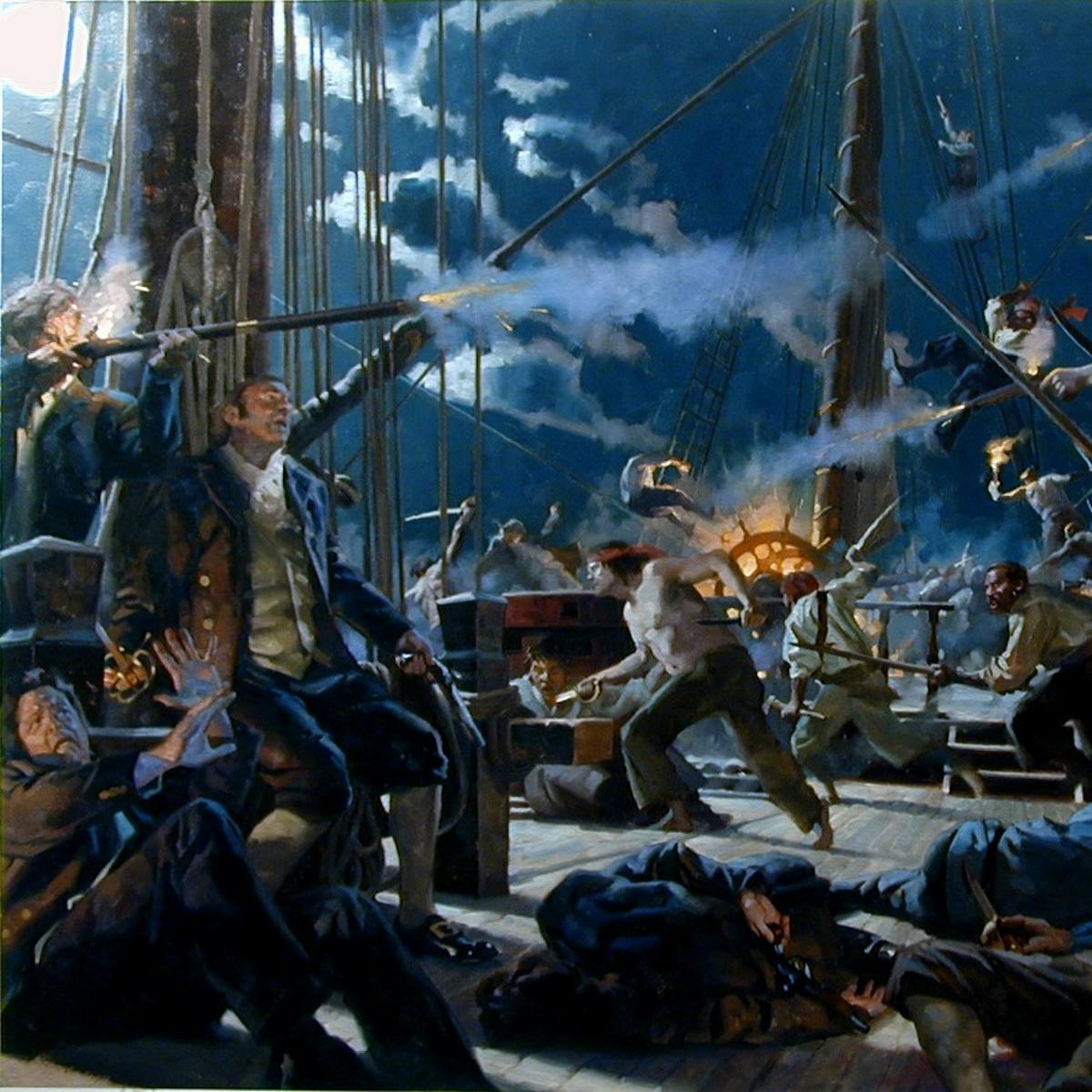The image is a detailed painting set at night of a dramatic and chaotic scene aboard a large sailing ship, possibly from the 1700s. The setting is illuminated by a full moon in a cloudy sky, creating a dark and gloomy atmosphere. Smoke from gunfire fills the air, highlighting an intense battle between sailors and pirates. The pirates, some shirtless and wearing dark colors with bands around their heads, are in the midst of attacking the ship, swinging from ropes and jumping onto the main vessel, possibly escaping a fire on their own ship as evidenced by red and yellow flames near a ship's steering wheel.

In the foreground, a British-looking gentleman in a blue uniform fires a blunderbuss, with sparks and smoke erupting from the barrel. Nearby, an injured man lies on the deck, while another, seemingly in defensive posture, raises his hands protectively. Amidst the chaos, another pirate stands menacingly with a weapon, and numerous injured or dead bodies are scattered across the deck. Diving deeper into the scene, a man hides next to a wooden barrel, seeking refuge from the onslaught. The artwork evokes a sense of historical realism, with intricate details capturing the harrowing and violent pirate attack on the ship.